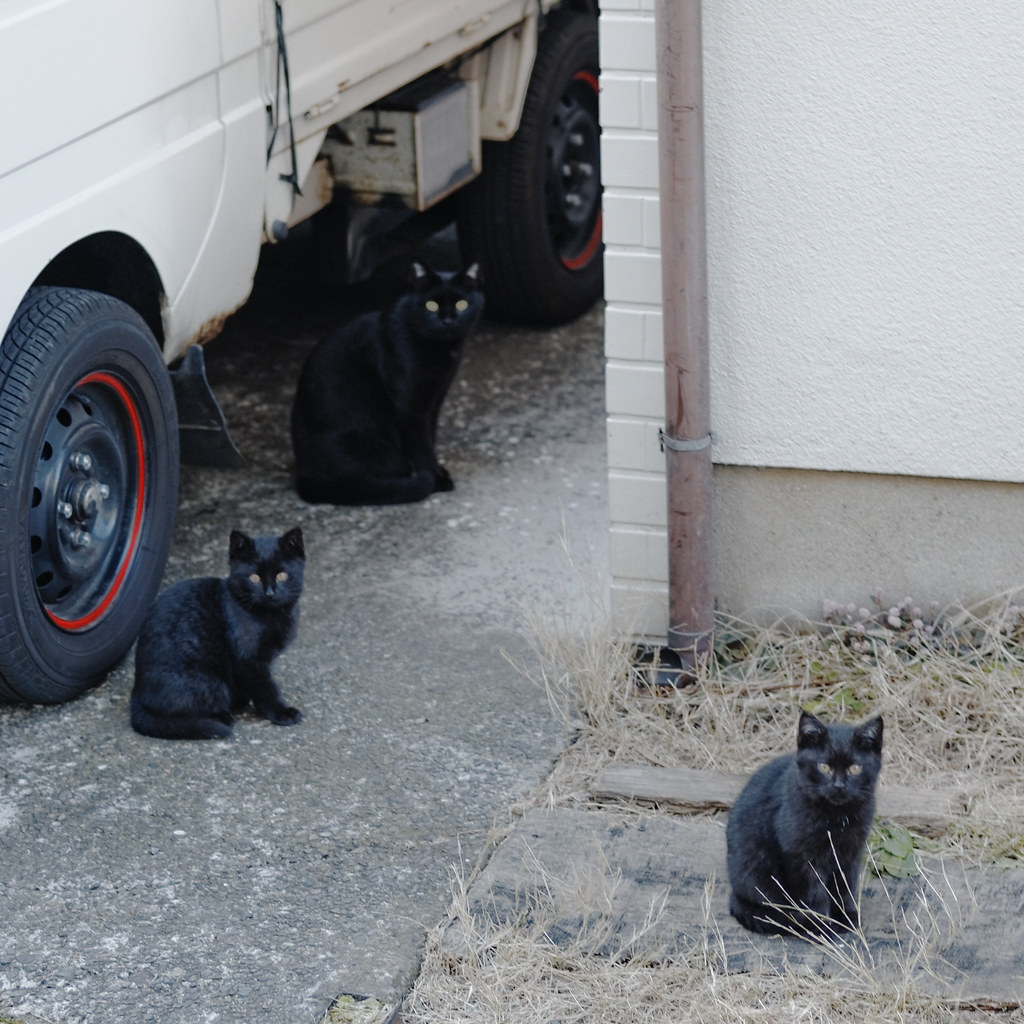In this detailed photograph taken outside near someone's home, there are three black cats positioned prominently in the image. Two of them, one larger with dark black fur and one a smaller kitten with dark grey fur, both with piercing yellow eyes, are sitting in front of a white truck with black tires and a red inner ring. The third kitten, also black and grey with yellow eyes, is positioned on a little pathway to the right and appears to be on dead grass. The backdrop includes a white wall with bricks lining it and a drain feature with an orangey-red ring. The entire scene exudes a sense of curiosity as all the cats are gazing directly at the camera, their vivid yellow eyes catching the light.